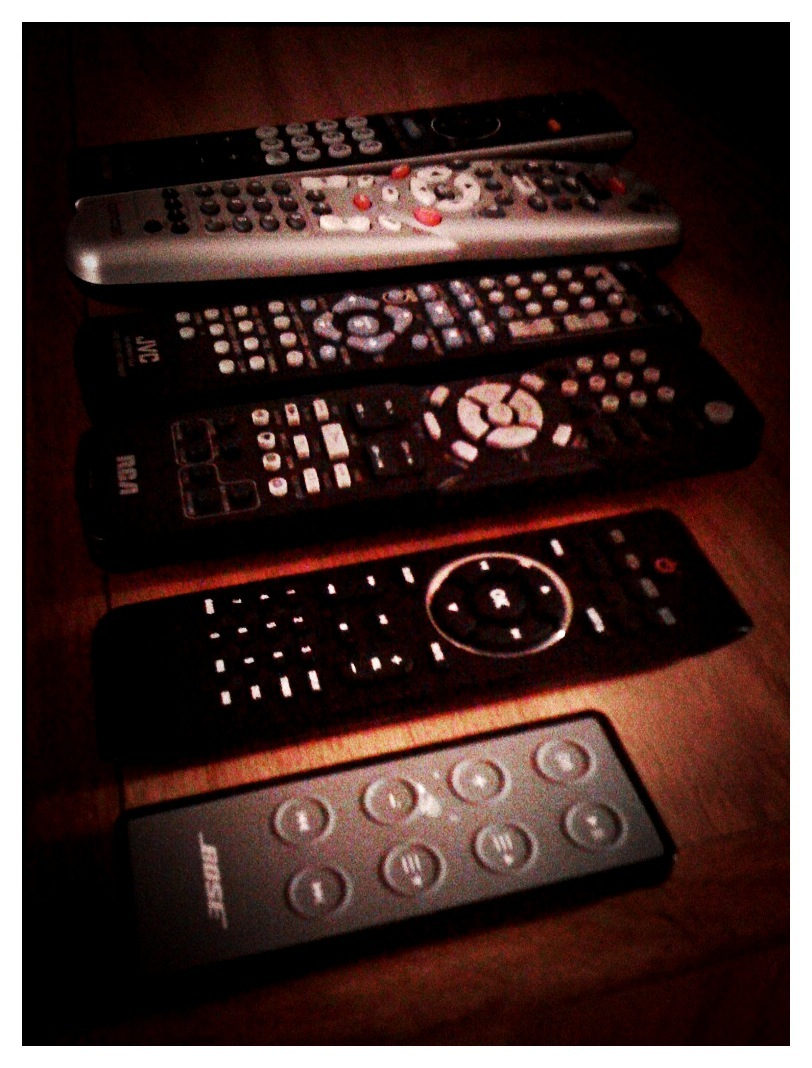This grainy, color photograph features an upright portrait orientation, reminiscent of a page from a book. Displayed on a wooden tabletop surface, six remote controls are meticulously arranged in a horizontal row. At the bottom of the image is a black Bose speaker system remote. Next to it, progressing left to right, is another black remote with indistinct labeling. The third remote, also black, is labeled RCA, typical of an RCA TV remote with white or gray buttons. Following the RCA remote is a black JVC remote. On top of the JVC, positioned in profile, is a slim silver-colored remote with dark gray, white, and red buttons. Completing the lineup at the top of the photograph is another black remote control. The photograph appears dark and shadowy, with a slight vignette effect, which adds to the detailed and somewhat mysterious presentation of these everyday objects.